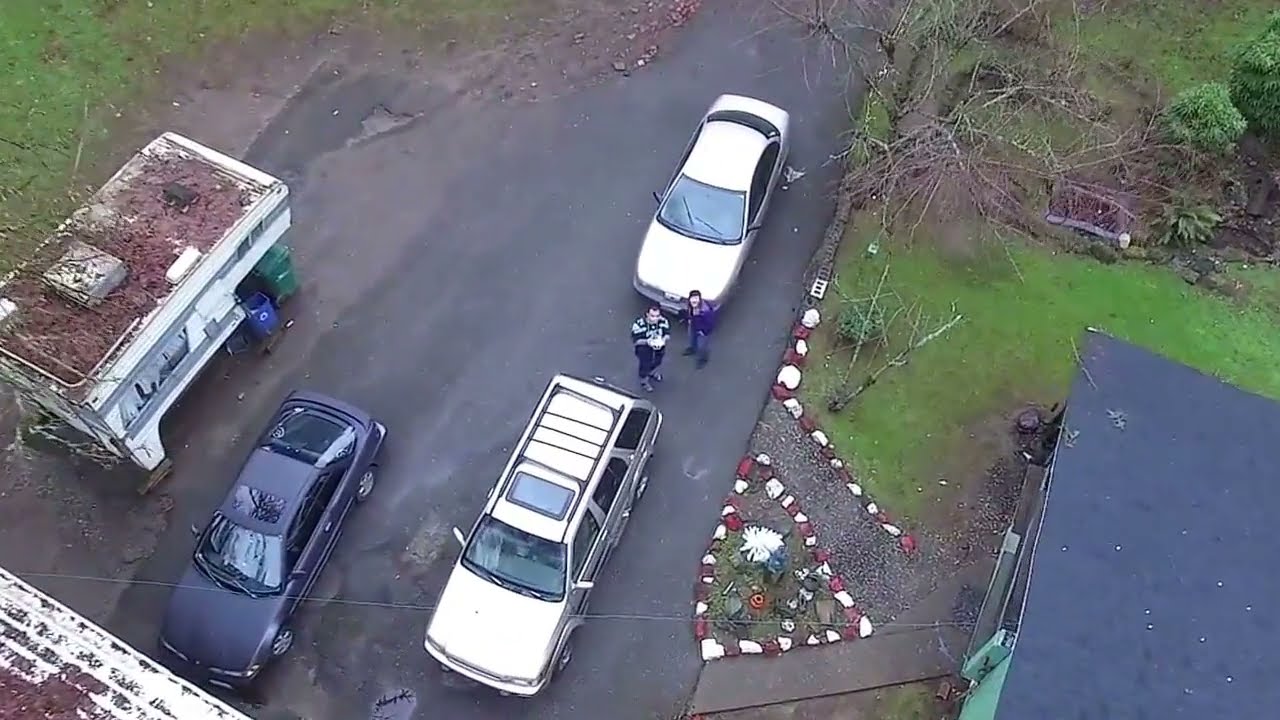This aerial image, likely captured from a drone, shows a detailed view of a driveway intersecting with a street. The driveway contains three parked vehicles: a silver sedan, a silver van, and a dark gray sedan. Between the vehicles, two individuals can be seen looking up at the camera. One person appears to be wearing a purple coat and blue jeans, while the other is clad in a dark short-sleeved shirt and seems to be holding a remote control, possibly for the drone taking the picture. Adjacent to the vehicles is an old, dirty trailer covered with accumulated dead leaves and housing a couple of garbage and recycling bins underneath.

The image also captures the corner of a house with a gray roof on the right. A cement walkway extends from the house to the driveway, lined with alternating red and white rocks, and surrounded by small lawn trinkets. The surrounding area features a grassy lawn with a few trees, bushes, and broken branches scattered on the ground. Some trees appear to be barren, with fallen leaves visible on the path beside the driveway, signifying the autumn season.